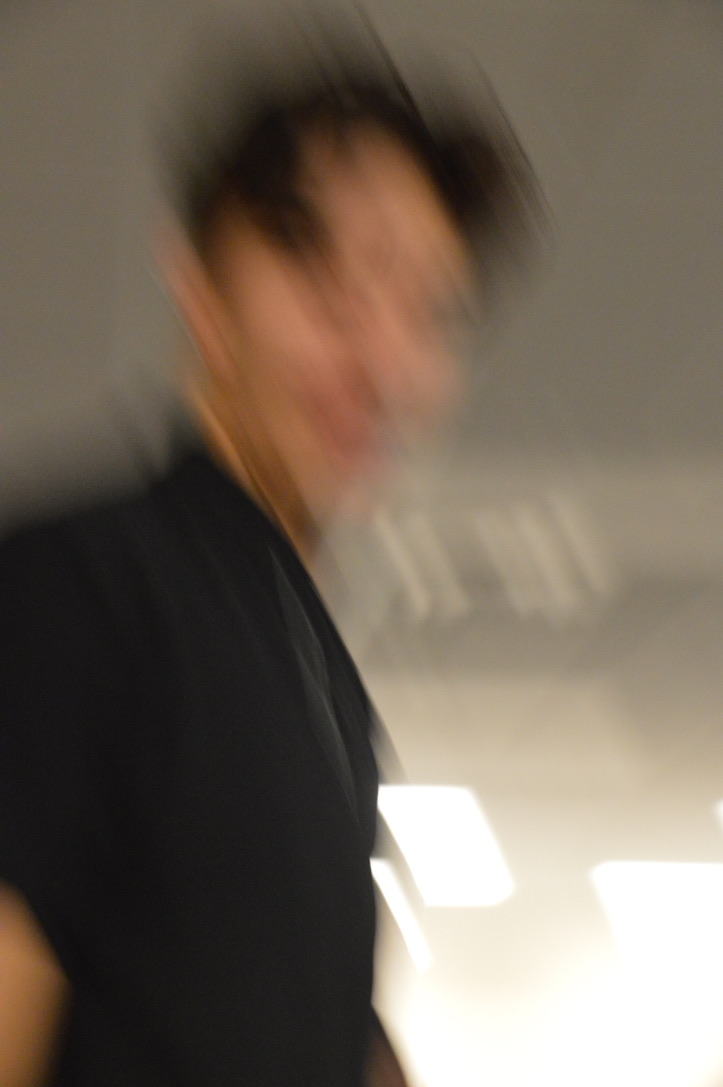A blurry portrait captures a man looking directly at the camera, with his smile subtly distorted by the out-of-focus effect. He is wearing a black short-sleeve shirt, and his wild, brown, receding hair stands out in the image. The gray background fills most of the frame, extending three-quarters of the way down, while the bottom right-hand portion is dominated by almost complete light with irregular shapes of light reaching up towards his chin, adding an unexpected brightness to the composition. Despite the blur, the man's gaze and smile convey a warm, approachable demeanor.